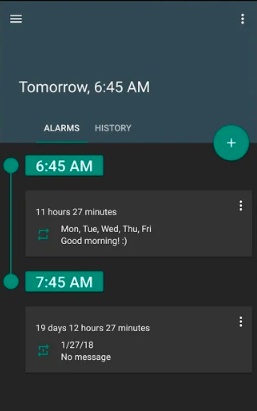A detailed caption for the image could be:

"Screenshot of an Android smartphone's alarm interface displaying multiple alarm settings. Near the top, in slightly off-centered white text, it reads 'Tomorrow 6:45 a.m.'. Below this are two tabs: 'Alarms' (highlighted in white) and 'History' (shaded in gray). The 'Alarms' tab is currently active. 

The first alarm is set for 6:45 a.m., displayed within a teal-colored box. Beneath this time, it indicates that the alarm is set to go off in 11 hours and 27 minutes, recurring on weekdays (Monday to Friday). Additionally, this alarm features a cheerful message, 'Good morning :)'. 

The second alarm is set for 7:45 a.m., and displays a countdown of 19 days, 12 hours, and 27 minutes until it activates, dated 1/27 and time-stamped 7:18. This alarm does not have any additional message associated with it."